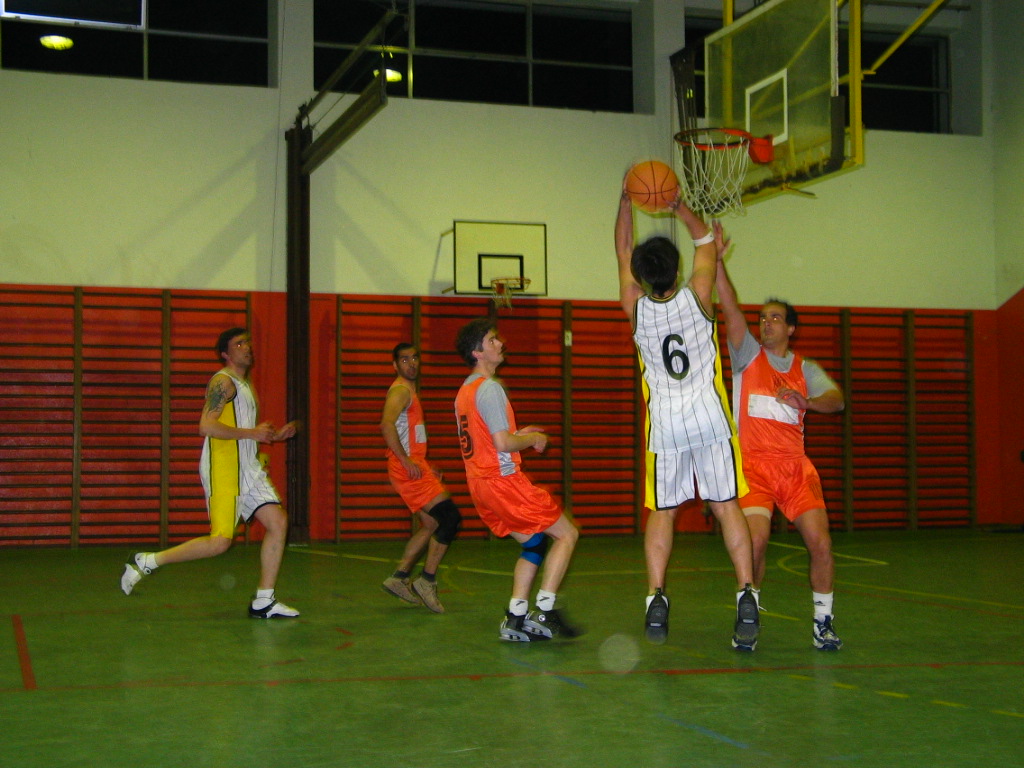This photo captures an intense moment during a men's basketball game at a recreation center. The setting suggests an amateur match rather than a professional showdown, highlighting the community spirit and passion for the game. Dominating the right side of the frame is a player in a white pinstripe jersey with yellow accents, numbered 6, captured mid-air as he attempts a crucial shot. His body is fully extended with the basketball poised above his head, feet suspended off the floor. In a defensive stance directly in front of him is an opponent in an orange tank top with a gray undershirt, striving to block the shot with his left arm firmly raised. To the left, two more players in orange jerseys are rushing towards the basket, adding to the dynamic energy of the scene. In the background, another player, possibly wearing the number 3 or 4, lingers, perhaps strategizing his next move. The tension and excitement of the game are palpable, encapsulating the raw enthusiasm of recreational sports.